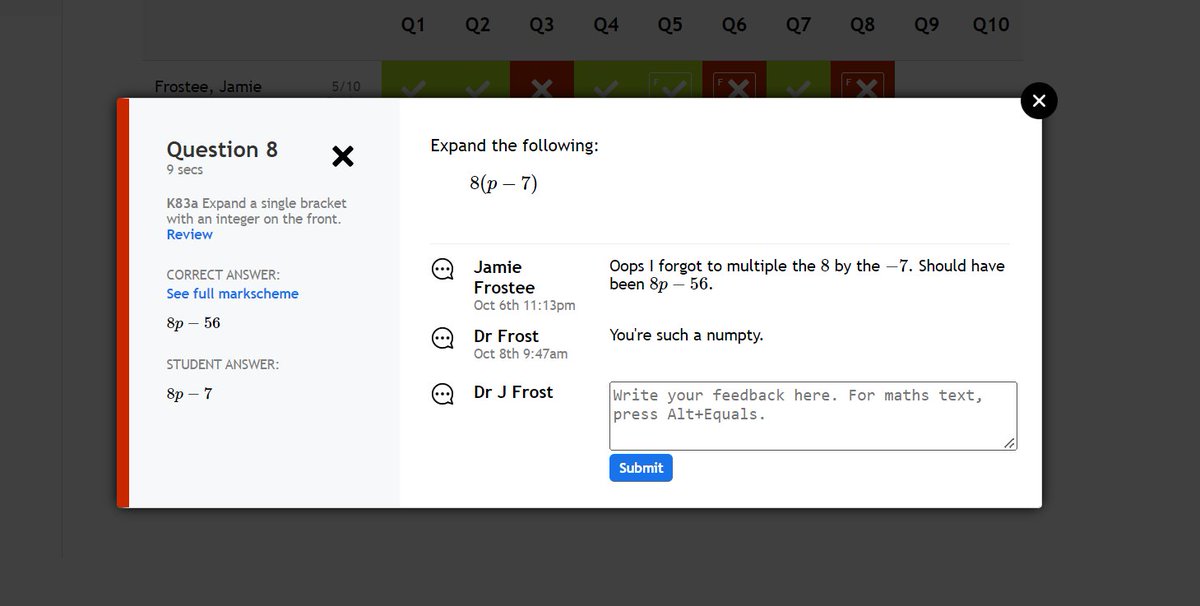The image depicts a computer screenshot with a grayed-out background. At the center of this background is a prominent window featuring a white backdrop filled with text. In the upper left corner of this white window is "Question 8," which is followed by a timer reading "9 seconds" and the code "K839." Below these identifiers, the instruction "Expand a single bracket with an integer on the front" is displayed.

The left vertical frame of the window is highlighted with a red border. Further down, beneath the initial instruction, the terms "Correct Answer" are written in blue, accompanied by "C4 Mac scheme."

On the right side of the window, there is a handwritten note stating, "Oops, I forgot to multiply. I forgot to multiply the 8 by the 7. It should have been 8P minus 56."